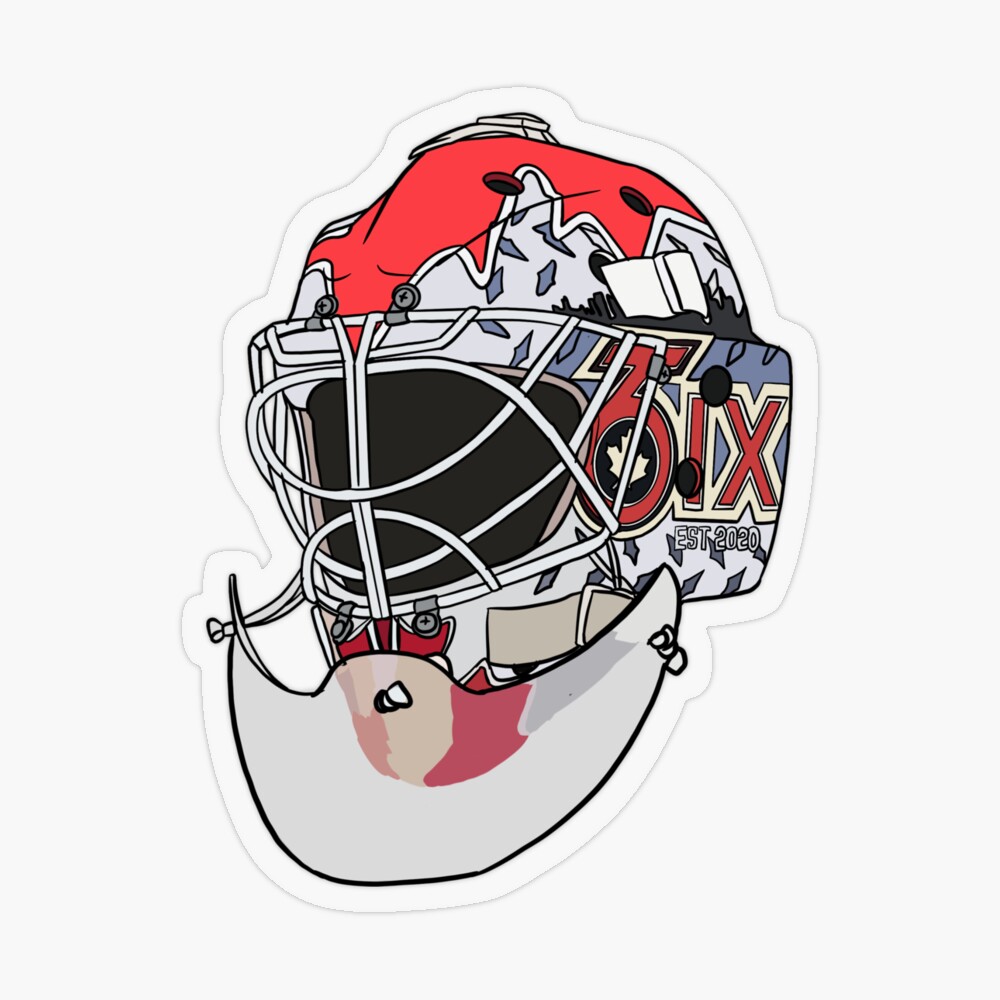The image features a professionally rendered, vertically rectangular depiction of a hockey helmet. It is primarily an off-white or very light gray with speckles of light purple throughout the helmet's surface. Dominating the top of the helmet is a large red streak interspersed with two ventilation holes. A white wire face cover is affixed to the front, which blends into a clear plastic mouth guard below.

Significant details include the numbers and text on the helmet, noting a distinct red "6" alongside "IX" in red on the side, along with a white maple leaf incorporated into the first number. Below this, in white text, are the words "ESTD 2020." The helmet is also outlined with gray trim and displays more small diamond-shaped polka dots at the bottom.

The image background is faint light gray, and the overall artwork appears to be designed without a border, suggesting the visual might be a sticker. The helmet’s intricate detailing and color scheme — particularly the red and white elements, alongside the protective face guard lacking a visor — contribute to the impression of a meticulously designed piece. There is no other text or objects present in the image.